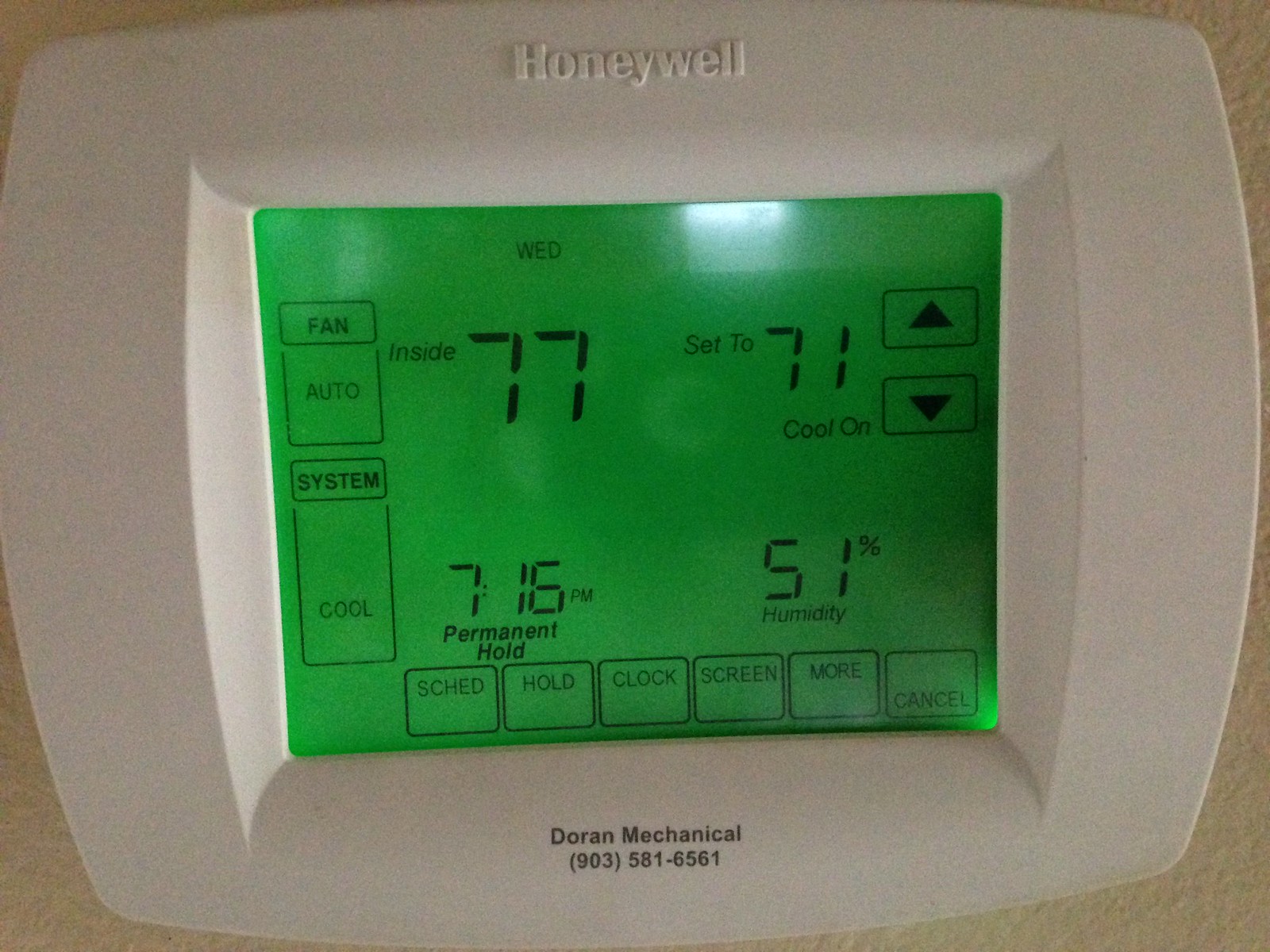This image features a Honeywell temperature control unit mounted on a beige or ivory-colored wall, with subtle shadowing enhancing the texture of the background. The unit is predominantly white with the "Honeywell" logo prominently displayed in raised letters. At the bottom of the unit is the label "Doran Mechanical 903-581-6561" in black print.

The digital display on the temperature control is backlit with a green hue, and it features black text for readability. The top of the display shows the day of the week, "WED," along with the time "7:16 PM." Key data on the screen includes the current indoor temperature, "77°," the set temperature, "71°," and the status "Cool On." Additionally, the display shows a "Permanent Hold" mode and indicates the indoor humidity level at "51%."

Control buttons on the thermostat include options such as "Fan," "Auto," "System," and "Cool," alongside operational buttons across the bottom for "Schedule," "Hold," "Clock," "Screen," "More," and "Cancel." There are also up and down arrows for adjusting settings.

This detailed depiction provides a comprehensive overview of the temperature control unit's appearance and functionality.